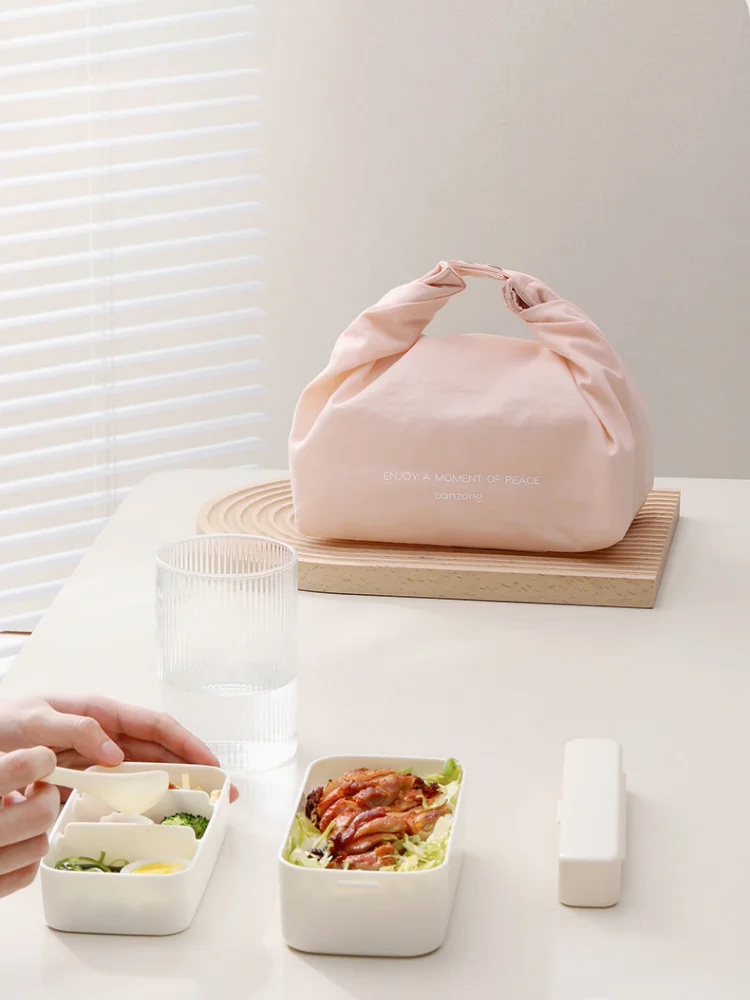The image is a realistic, close-up photograph featuring a variety of objects arranged on a white table in a white room. At the bottom left corner, a pair of white-skinned hands are seen eating from two small white trays using a white spoon. The trays contain various foods, including meat, lettuce, and a boiled egg. To the foreground, there's a large, textured glass of water, half-full, positioned slightly behind and to the right of the hands. Further to the back, a rectangular box wrapped in a faintly lettered pink cloth rests on a wooden cutting board. The cutting board is about an inch thick, 12 inches long, and 6 inches wide, with a rectangular bottom and a semi-circular top, featuring slight linear designs. On the far right, there appears to be a stick of butter or another small closed tray. The overall scene is set against a clean, white background.